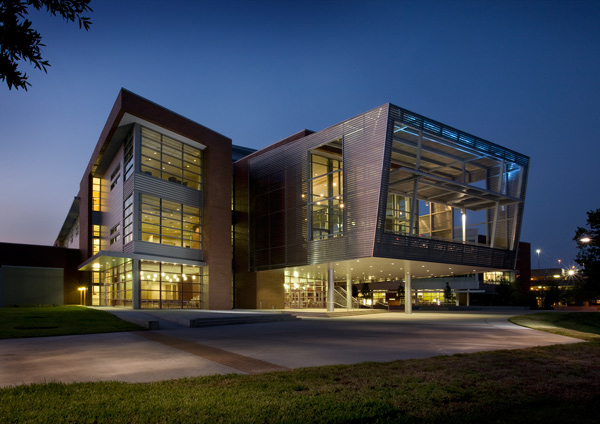The image captures a strikingly modern three-story building at night, characterized by its sharp architectural edges and abundant windows that flood the interior with light. The building, possibly an office or a sophisticated library, features a two-level balcony and a distinctive cage structure jutting from its front. Floor-to-ceiling windows on the left side provide a transparent view inside. The exterior includes a concrete driveway, a sidewalk, and a manicured lawn, blending urban design with nature. Surrounding the building, the scene extends to street lamps, a paved access road, and glimpses of other structures on the right-hand side. The scene is set against a dark blue sky that transitions into a subtle yellow gradient near the horizon, suggesting the sun has recently set.